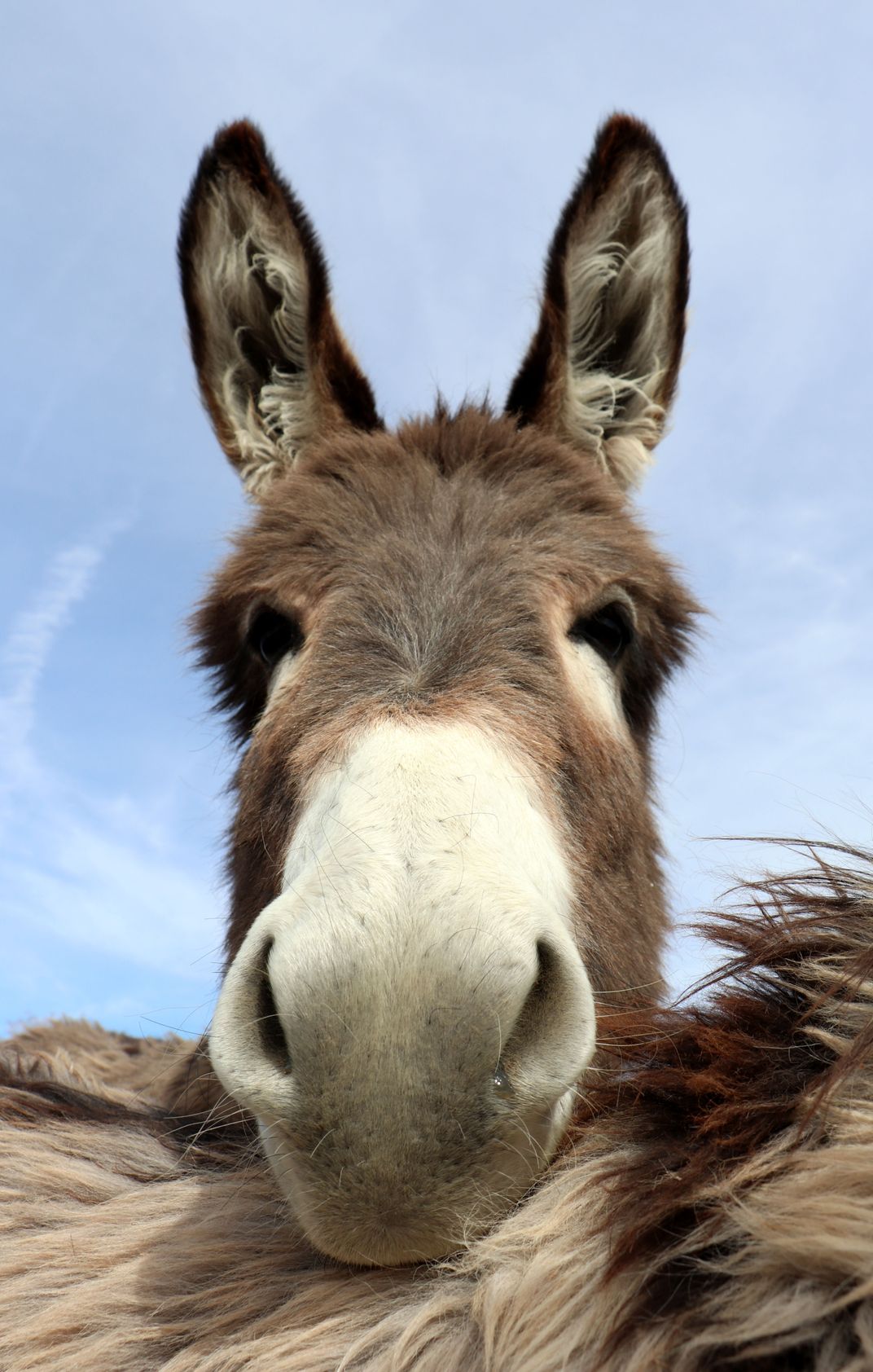This is a vertically-oriented image featuring a close-up of a donkey's face, positioned front and center. The donkey's sizable white snout with flared nostrils and its dark brown fur covering most of its face, including around its cheeks and eyes, are prominent. Its tall, erect ears are brownish on the outside and lined with white on the inside. The donkey appears to be resting its head on what seems to be another animal with a similarly colored coat, primarily light cream and chestnut brown. In the background, the sky is a light blue adorned with wispy white clouds, adding a serene atmosphere to the scene. The donkey's eyes, almost black, gaze directly at the viewer, adding a sense of connection to the image.